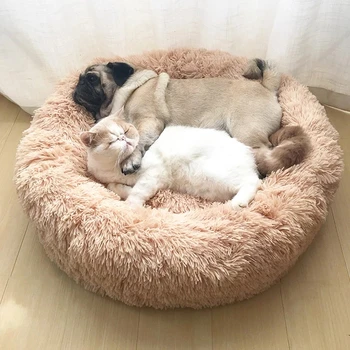The image depicts a cozy scene of a light brown, donut-shaped pet bed with a hint of pink, sitting on a light brown hardwood floor. Inside the fluffy bed, a pug and a cat are nestled together. The pug, with its characteristic black snout, curled tail, and tan body, has its left arm gently wrapped around the cat. The cat, a white-furred feline with brown ears and a tail, has its eyes closed, appearing content and relaxed. The setting includes a white curtain in the background, providing a serene backdrop for this affectionate display, with no other objects visible in the room.